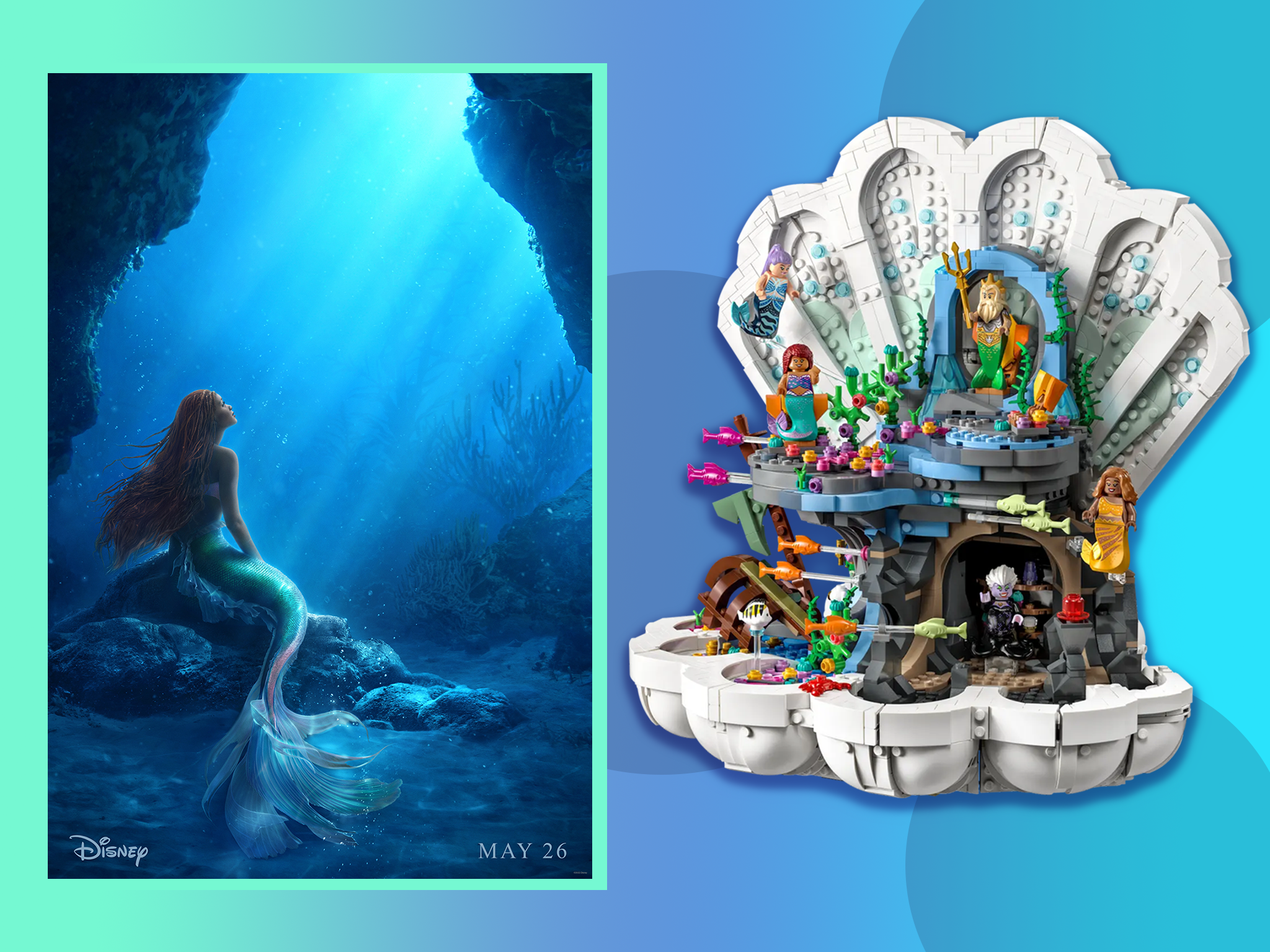This image is composed of two distinct pictures side-by-side. The first picture is a promotional poster for Disney's new Little Mermaid movie featuring the African-American Ariel. In this underwater scene, Ariel, with her long reddish hair flowing, is seated on a rock with her fins trailing behind her. She gazes upwards at the sunlight streaming through the water. The word "Disney" is displayed in white letters in the bottom left-hand corner, and the release date, "May 26," is shown in the bottom right-hand corner. The second picture is a constructed Lego set themed around Disney's Little Mermaid. This set is vibrant and colorful, featuring a large white clamshell as the backdrop. Inside the clamshell, a merman holding a trident is visible, alongside a Lego figurine of Ariel, another mermaid, and a fish. Diverse colors, a treasure chest, and a blue background complete the undersea tableau, creating a vivid and eye-catching display.